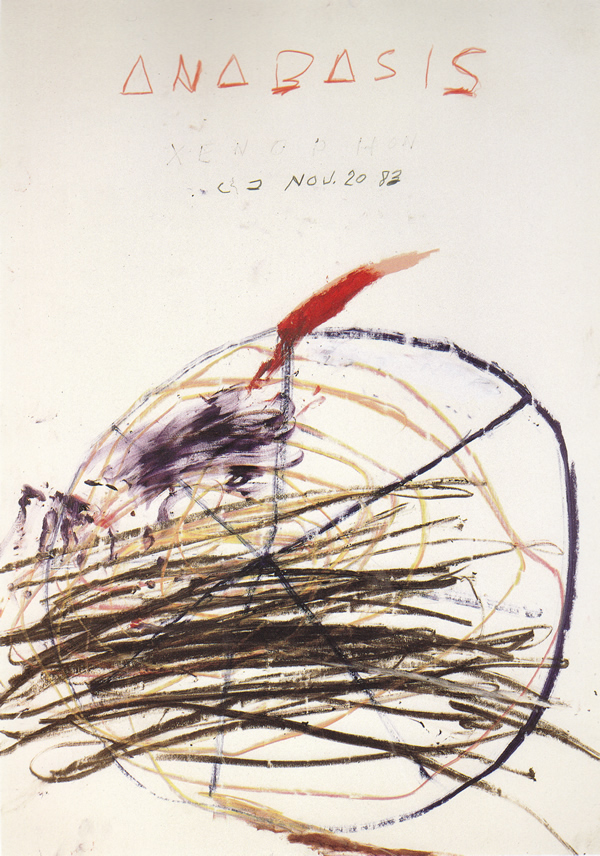The image features an abstract, child-like artwork executed in a mixture of crayon and possibly oil pastel on a beige or off-white background. The focal point is a black circular figure, divided into six segments resembling a spoked wheel or snowflake, positioned towards the bottom half of the vertical rectangular canvas. This central figure is heavily overlaid with various thick and thin scribbles and smudges, predominantly in dark gray or charcoal, and a prominent red streak that protrudes from the top, resembling a flame. Surrounding this structure are random streaks and smudges in colors including purple, brown, yellow, tan, white, and orange, adding layers to the chaotic yet intriguing composition. At the very top of the image, there is text written in a Greek-like style that reads "ANABASIS" followed by "C2 NOV 2083," suggesting a date—November 20th, 2083.